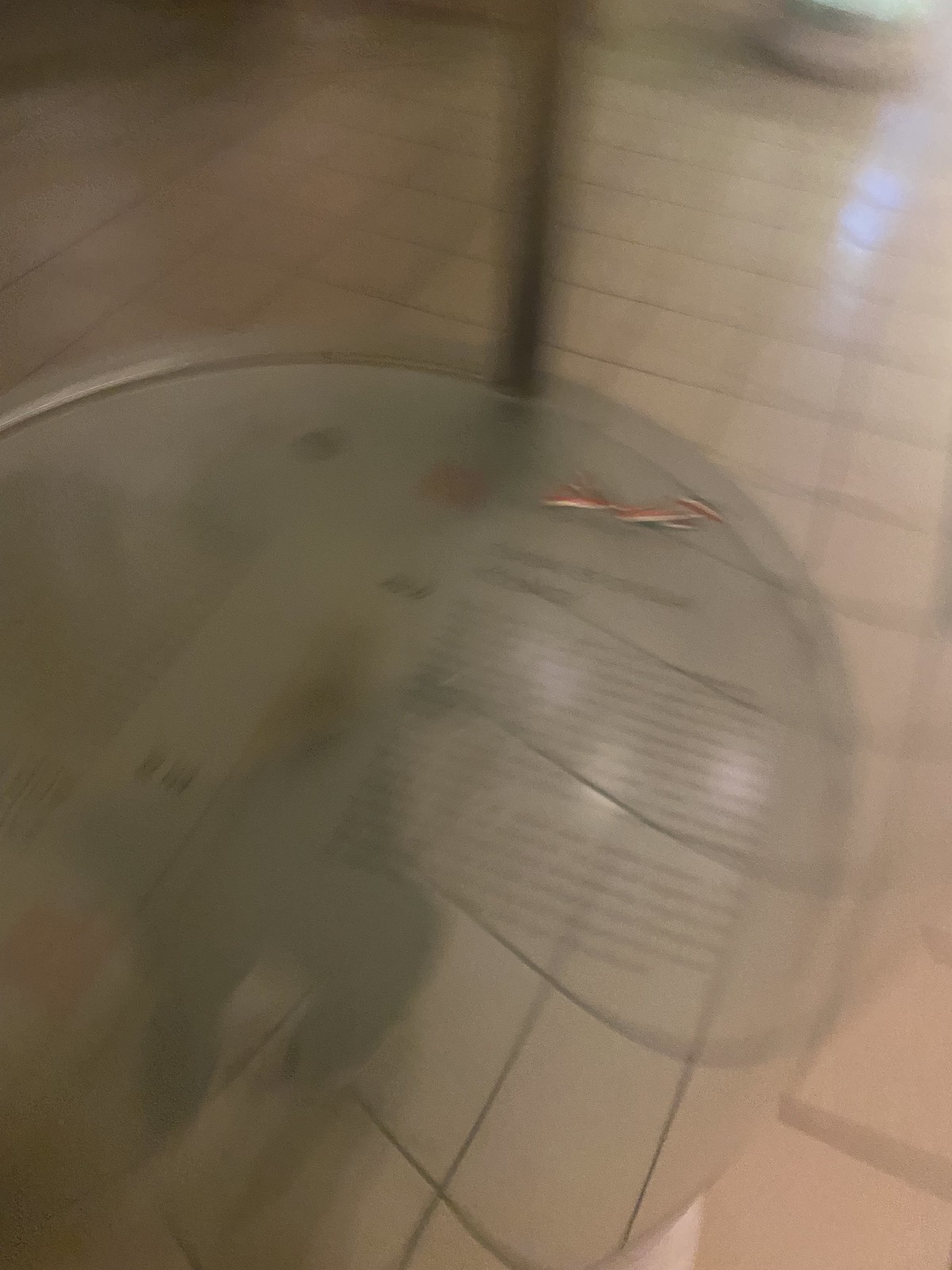The image is a portrait-oriented, extremely blurry photograph taken indoors. It primarily features a very shiny, square, white tiled floor with grey or black grout in between the tiles. The tiles are clearly visible but distorted through a central, transparent, circular object that occupies the lower two-thirds of the image. This object could be a glass panel or possibly a mirror, as the reflection of the floor tiles and a ceiling lamp can be seen on its surface. Extending from the center of the image upward, there is a blurry pole that appears to be metal. The circular panel on the object features some unreadable text, possibly serving as an information display, suggesting that this might be in an exhibition setting. Light reflections are present, possibly from a nearby window or other light source.